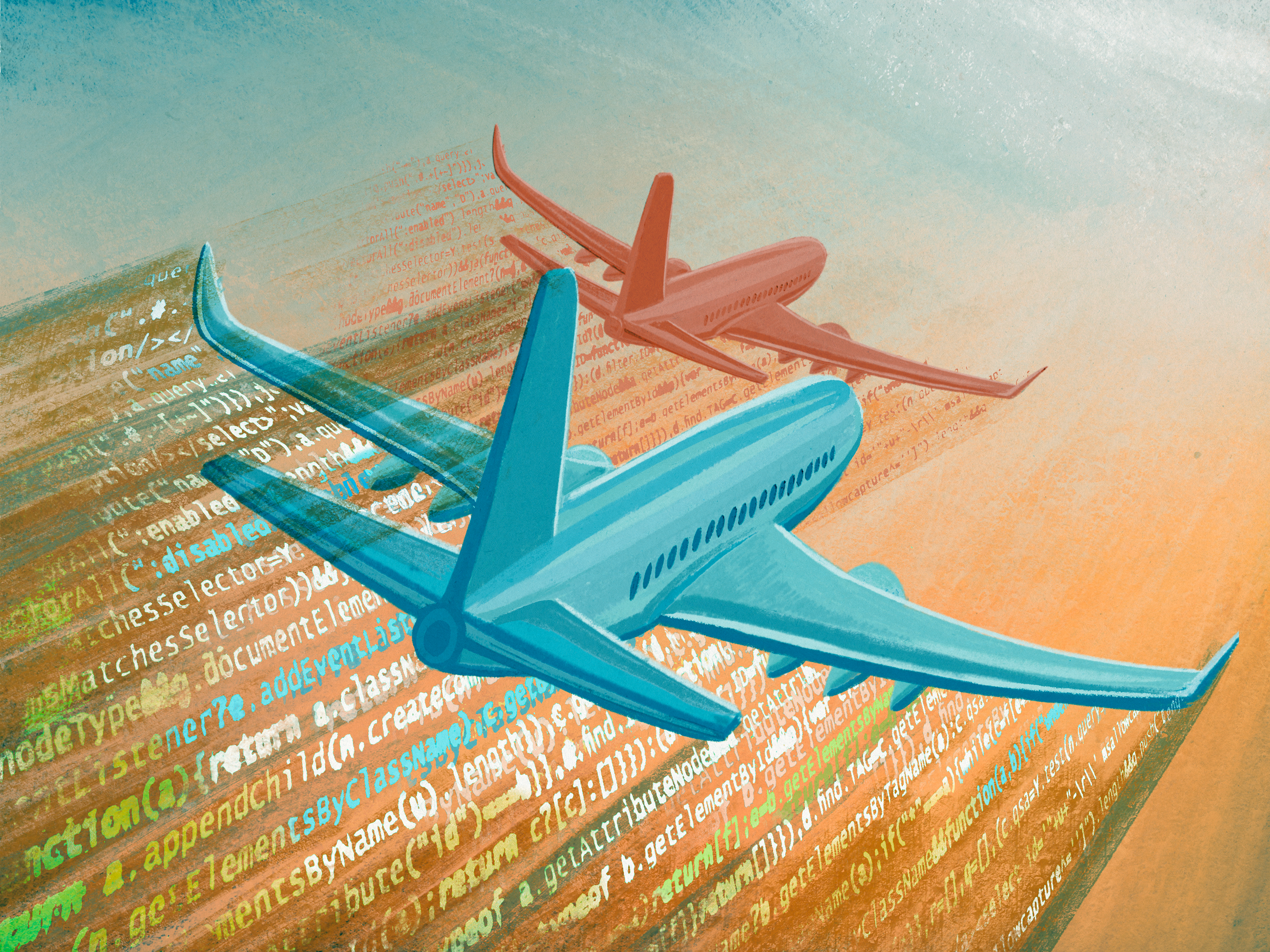This vibrant painting depicts two passenger jet planes soaring high in the sky. The leading plane, painted in a rich pink hue, features three engines on either side and fully extended wings that curve upward towards the tips. Closely following behind, the trailing plane is an aqua blue color, identical in structure with numerous passenger windows and similarly curved wingtips. Both planes appear slightly tilted, giving the impression of a gentle turn. Distinctively, instead of the typical contrails, streams of colorful computer code—from languages like Python, C-sharp, or C++—trail behind them, creating a striking visual contrast to the clear sky. The code streams are in vivid shades of yellow, green, blue, and white, further emphasizing the digital, surreal nature of the scene. The overall composition hints at a computer-generated aesthetic, enhanced by the unrealistic yet captivating representation of the aircrafts and their unique jet streams.